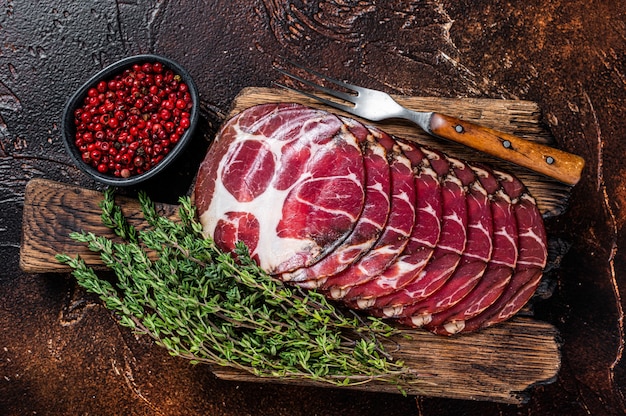In the image, an overhead shot captures a rustic charcuterie board displayed on a roughly finished concrete countertop that exhibits shades of brown, black, and tan. The charcuterie board itself is crafted from a jagged, dark-colored piece of walnut lumber, resembling a natural, carved piece from a tree or possibly a broken-off piece of a ship. On this rich, wooden board lies a vivid arrangement of sliced red and white meat, meticulously organized. Adorning the display, three or four sprigs of rosemary serve as a decorative touch.

To the top left of the board, a small, round black bowl brimming with whole cranberries sits, adding a pop of vibrant red to the spread. Close by, a distinctive three-tined fork, notable for its long metal prongs and medium-toned brown wooden handle accented with three round silver screws, rests on the edge of the board, waiting to be used. This detailed arrangement provides a visually appealing and inviting scene, perfect for a culinary delight.